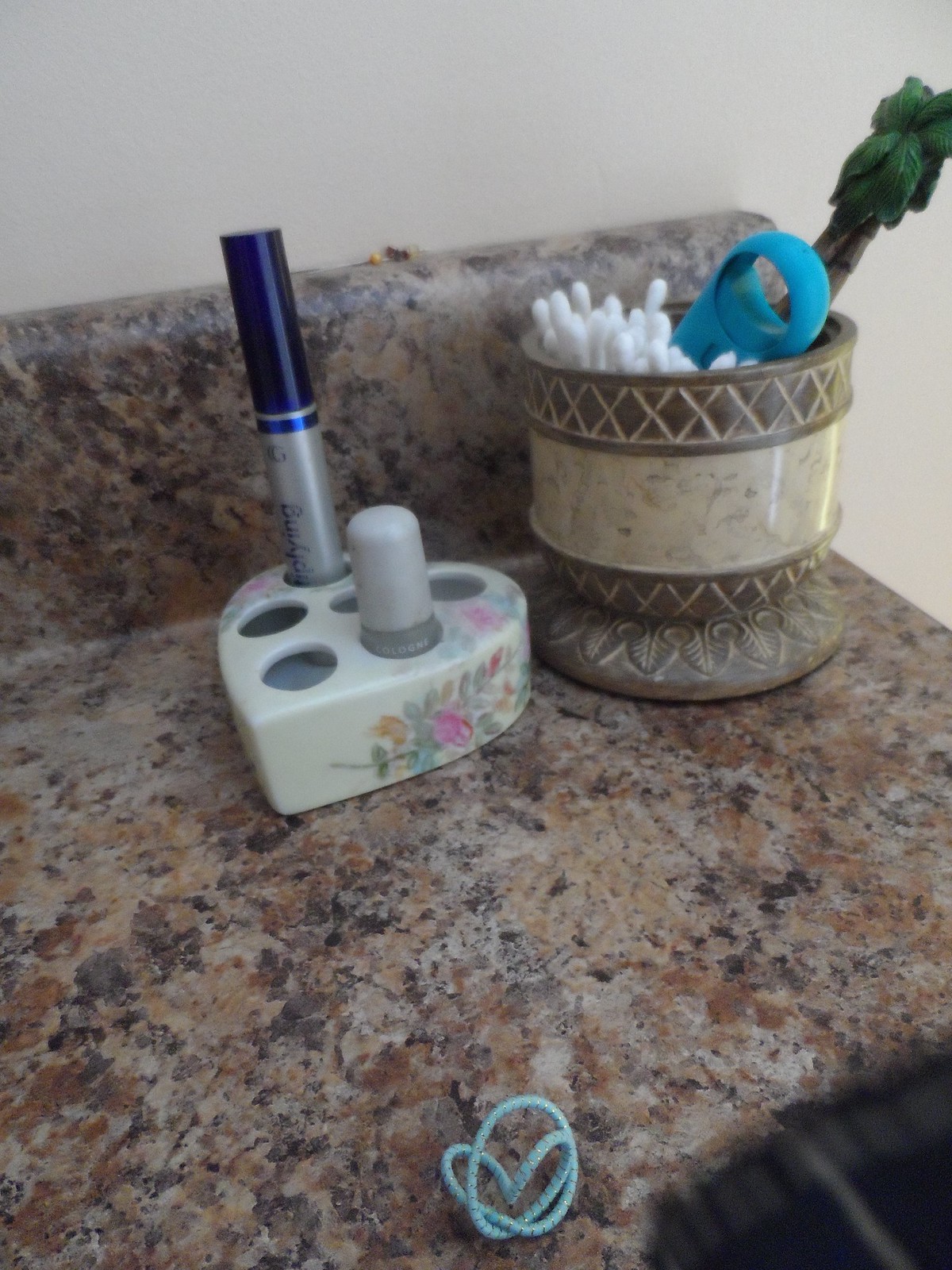This close-up image captures a segment of a bathroom countertop with meticulous detail. The countertop itself is visible in the lower and upper portions of the image, showcasing a brownish-mauve hue. In the bottom center, there's an aqua blue hair tie, scrunched up and casually placed.

Positioned prominently in the upper center are two containers. The first is heart-shaped and white, featuring six holes designed to hold items upright. Currently, it contains mascara and lip gloss in two of these holes, leaving four vacant. Next to it stands a unique cup filled with Q-tips. This cup is adorned with a tree-shaped accessory, cleverly integrated to serve as a handle. A small glimpse of the black background and the base of the countertop frames this orderly scene, further highlighting the organized yet intimate setting of this bathroom counter.